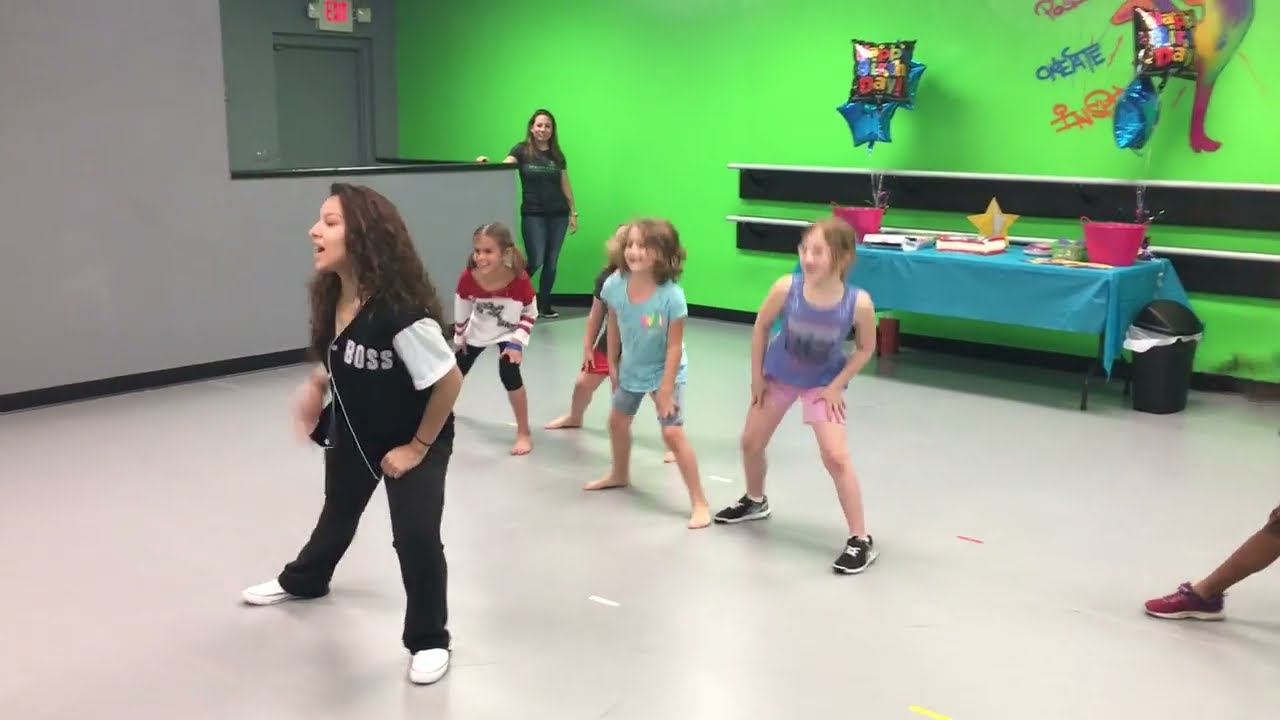In a brightly decorated event space with vibrant lime green and plain gray walls, a dance instructor is leading a dance lesson for four young girls, likely around eight or nine years old. The floor is a light gray terrazzo or cement, adding to the modern feel of the room. The instructor, a woman in her early 30s with light brown skin and long curly brown hair, is wearing a black baseball jersey with white sleeves, black pants, and white tennis shoes. She is crouched slightly, with one knee bent and her chin up, demonstrating a dance move. The girls, three of whom are barefoot, are lined up behind her, trying to mimic her movements. Each girl is dressed casually; one is in a red and white t-shirt with black leggings, another in a gray shirt with red shorts, the third in a blue shirt, and the last girl's details are not visible. In the background, a table with a blue tablecloth and balloons spelling out "Happy Birthday," along with visible cake and snacks, suggest a birthday party event. A mom with long brown hair stands near a door, watching the girls enjoy their dance lesson. This setting appears to be a versatile event center where birthday parties and dance lessons can be held simultaneously.